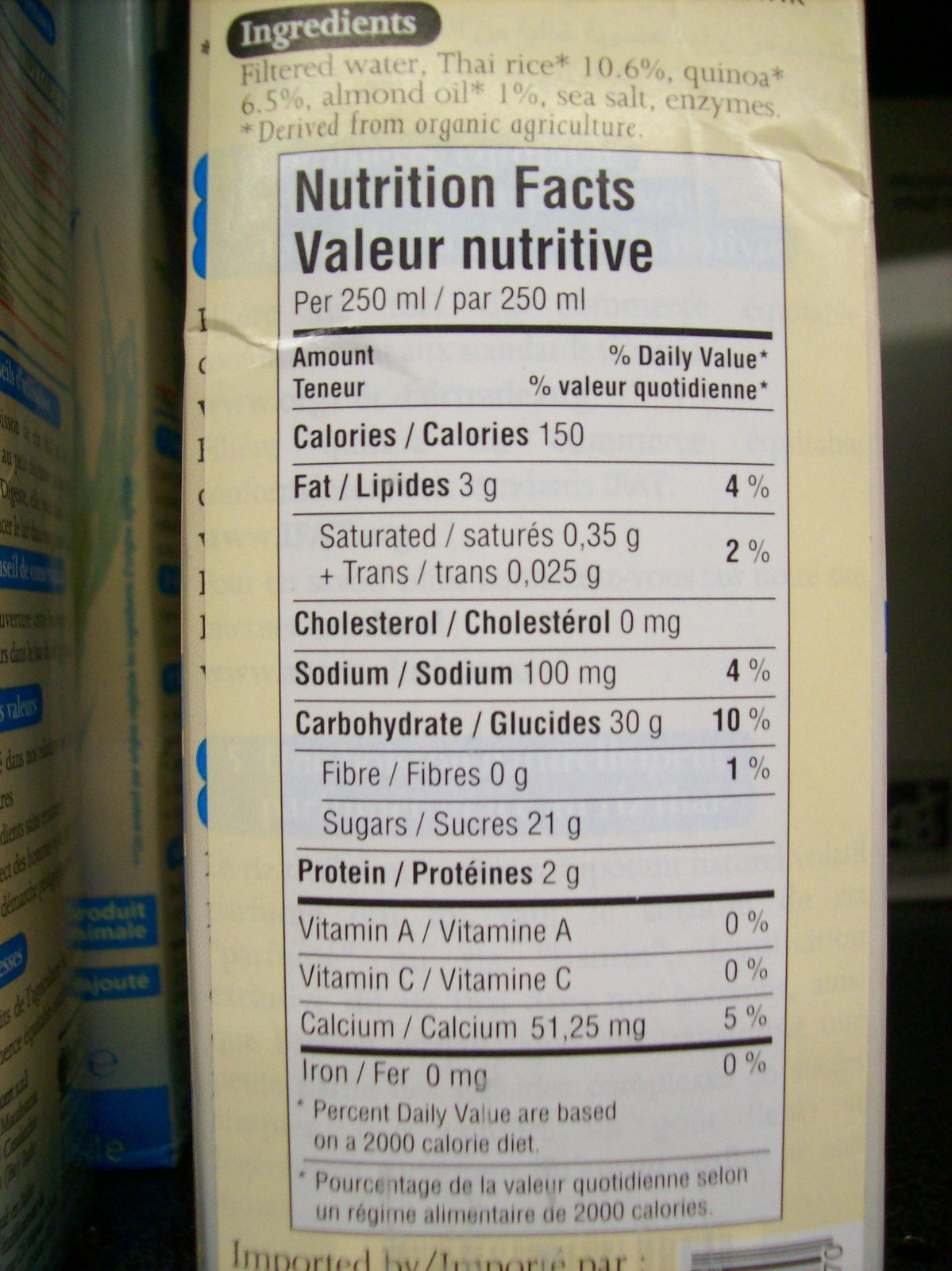This image captures a detailed view of the nutritional information on the side of a pale yellow carton of food, taken from a side angle. The carton features a prominent white Nutrition Facts label with black text, enclosed within chocolate brown dividing lines. Key ingredients listed are filtered water, Thai rice (10.6%) derived from organic agriculture, quinoa (6.5%), almond oil (1%), sea salt, and enzymes. The nutritional details provided include values for a 250 milliliter serving: 150 calories, 3 grams of fat (4% DV), 0.35 grams of saturated fat (2% DV), 0 milligrams of cholesterol, 100 milligrams of sodium (4% DV), 30 grams of carbohydrates (10% DV), 0 grams of fiber (1% DV), 21 grams of sugars, 2 grams of protein, 0% Vitamin A, 0% Vitamin C, 5% Calcium (51.25 milligrams), and 0% Iron. The information is presented in both English and French, hinting that the product may be European, possibly French. The carton’s aesthetic is complemented by a cream-colored background, adding to its visual appeal.